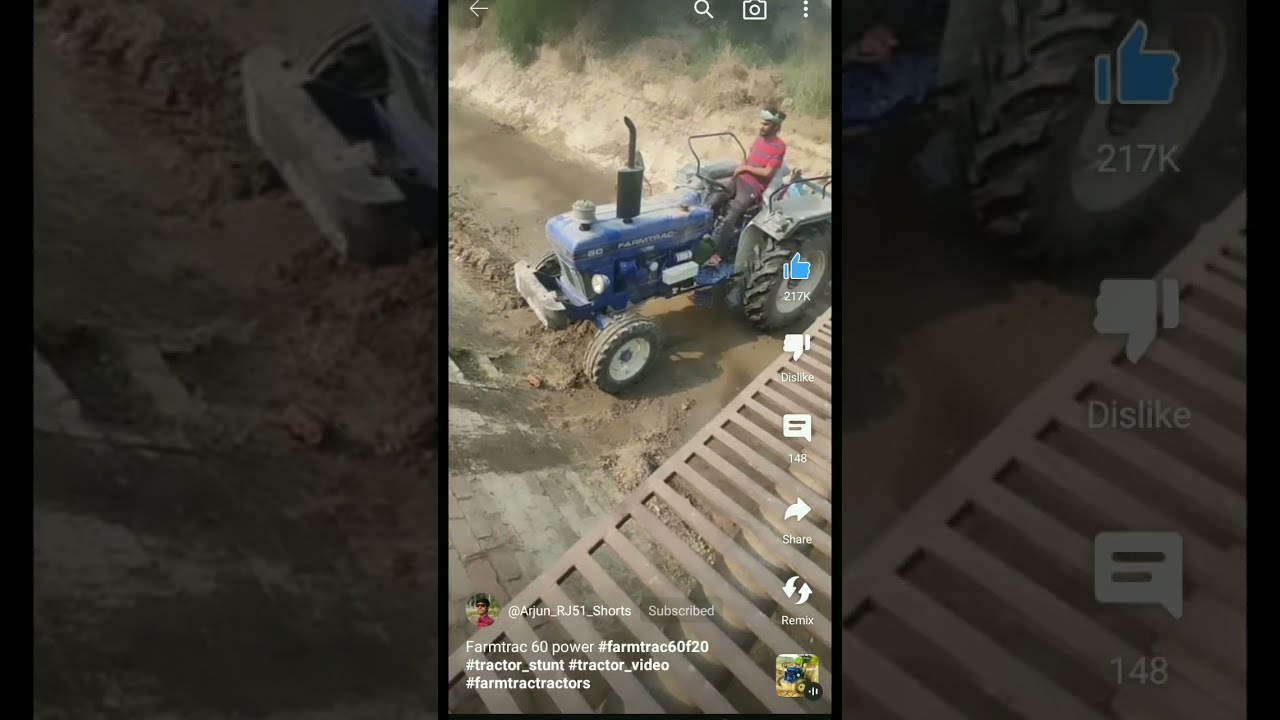The image is a vertical screenshot from a social media post, showing a man on a blue tractor at the bottom of a mostly dry, muddy canal. The man, wearing a red shirt and a headband of blue or white, seems to be navigating or idling the tractor by a dirt road flanked by brick embankments. The scene is viewed from an elevated metal walkway, almost like a grate, about 10 feet above. Surrounding the main image, the background consists of zoomed-in and faded sections of the same picture, creating a landscape frame. On the right side of the post are various interactive icons—like, dislike, comment, share, and remix—suggesting a common social media format, possibly Instagram. At the bottom, there's an avatar with a handle indicating that the user is subscribed, accompanied by text reading "farmattract60power" and several hashtags like #farmattract60f20, #tractor_stunt, #tractor_video, and #farmattractors.